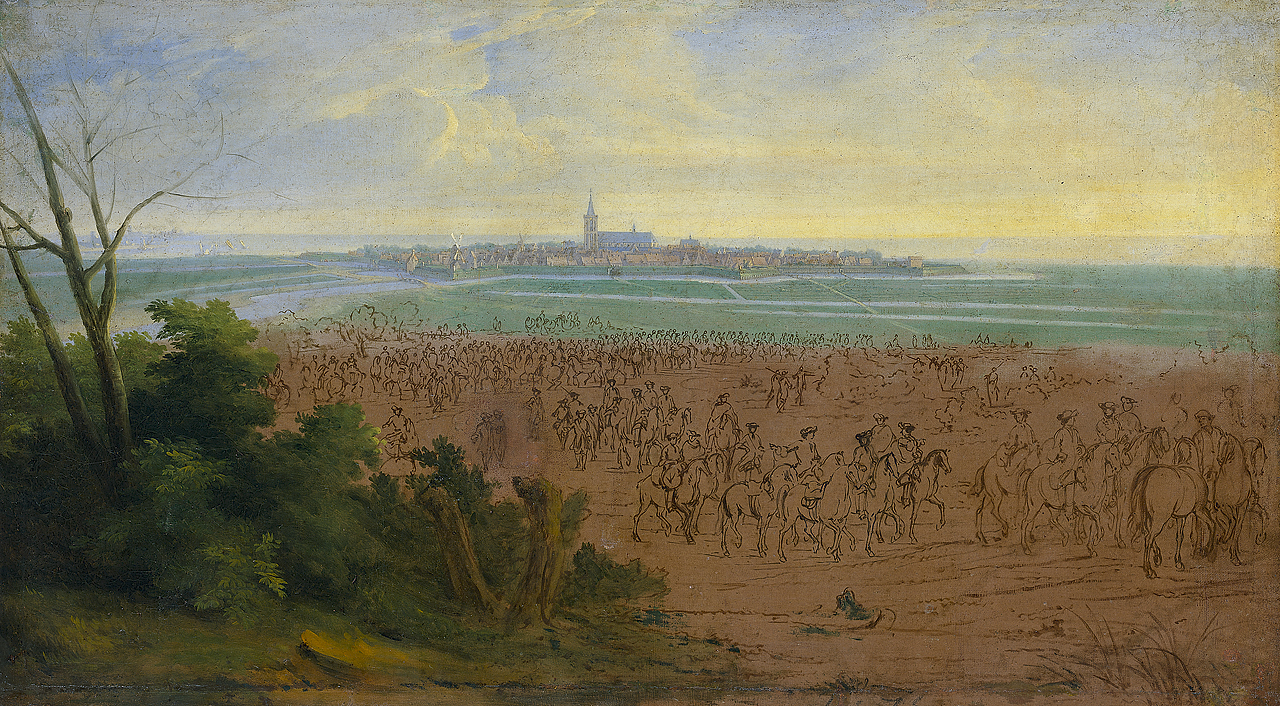This painting, likely by Frantz van der Meulen titled *Troops of Louis the 14th*, depicts a detailed landscape. The foreground features a large, flat expanse of brown ground with various lines suggesting it is dirt or undeveloped terrain. Scattered over this area are detailed yet incomplete line sketches of numerous soldiers and horses, appearing like unfinished black pen drawings, indicating the artist's intention to illustrate troops marching or preparing for battle without fully coloring them in. To the left, there are patches of green shrubs and a bare tree without leaves, providing contrast to the barren ground. Beyond this foreground, a body of water extends towards the horizon, where an island appears, housing a quaint building with a prominent steeple, possibly a church. The sky above is a mix of blue with heavy clouds gathering near the horizon, some tinged with yellow hues, perhaps hinting at dawn or sunset. The scene captures the juxtaposition of nature, human activity, and architectural elements in a harmonious yet somewhat unfinished composition.